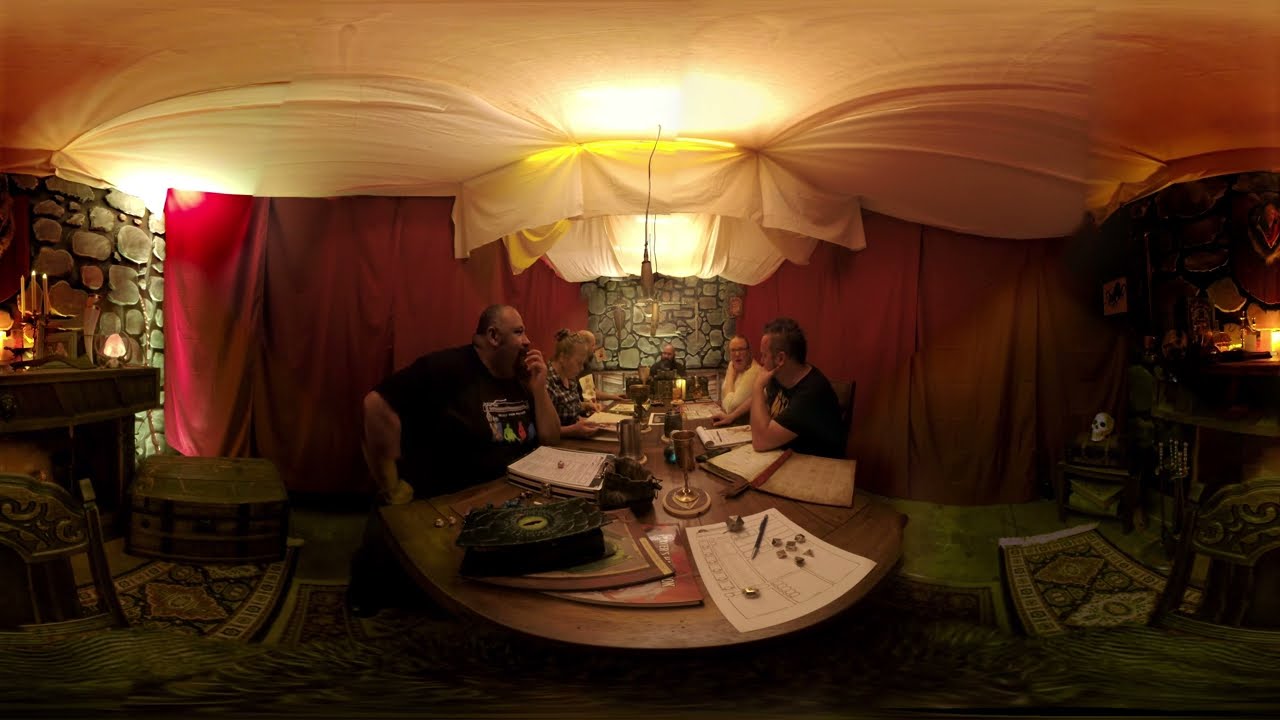The image depicts a dimly lit, medieval-themed restaurant interior with a fisheye perspective, giving a slightly warped view of the room. At the center, a large dark brown wooden table is surrounded by people, some wearing black shirts. On closer inspection, these individuals appear to be engaged in a tabletop game, possibly Dungeons and Dragons, as suggested by the presence of books, notebooks, white paper with pens, and dice scattered across the table. The setting is adorned with intricate details: red curtains hang against a gray stone wall in the background, which also features a fireplace with candles on the mantelpiece. Rugs with floral designs embellish the floor. The ceiling is draped with white fabric, creating the appearance of a canopy, adding to the room’s medieval charm. Golden chalice-like drinks adorn the table, enhancing the thematic ambience. Multiple people, including some women, are present, contributing to a lively, immersive atmosphere.